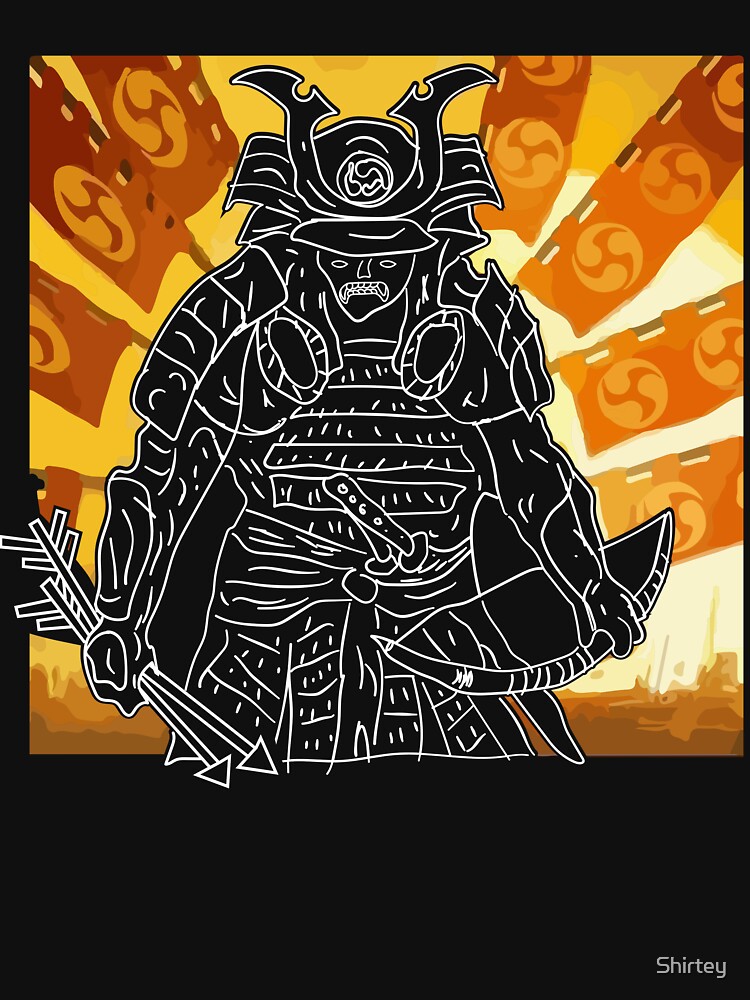This detailed, comic-style artwork features a menacing samurai warrior in black and white, accented with white outlines. The samurai dons a horned helmet with two prominent horns pointing out to the sides and has a stern, angry expression characterized by narrow, beady eyes, a simple square nose, and a sharply defined mouth with pronounced jaws. He wears heavy, intricate armor on both arms, with a recurved bow grasped in his right hand and two arrows in his left. A sword is sheathed at his waist, angled downward to the right.

The iconic warrior stands against a vibrant background dominated by a bright sun and radiating orange, yellow, and red hues. This sunburst pattern is enhanced by flags that emanate outward like rays, each flag featuring circular designs reminiscent of Chinese stars or fidget spinners. The image is bordered by a thick black band at the bottom, thinner black borders on the top and sides, and inscribed in the bottom right corner with the artist's signature, "SHIRTEY," in gray or white lettering. The entire ensemble creates a striking contrast, setting the monochrome samurai against the vivid, colorful backdrop.